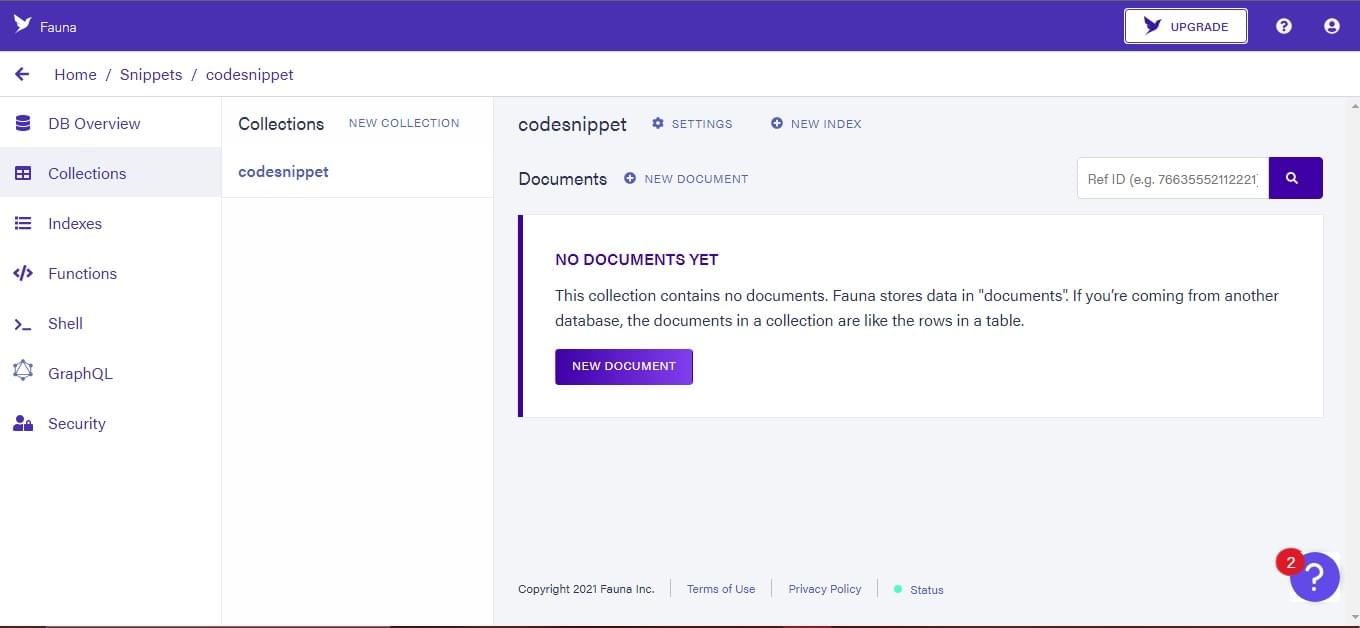The screenshot depicts a navigation window primarily designed in white, accented with light gray sections and purplish dark blue details. Dominating the top is a purple bar with a bird icon and the text "Fauna." The top right corner features three buttons: one for upgrading, a question mark, and a circular profile icon. Below this bar, the navigation options are displayed in two columns.

On the left-hand side, a vertical menu lists options in descending order: DB Overview, Collections, Indexes, Functions, Shell, GraphQL, and Security. The 'Collections' option is highlighted, leading to a sub-menu with 'Collections,' 'New Collection,' and 'Code Snippet.'

The main body of the window under 'Code Snippet' displays three tabs: 'Code Snippet,' 'Settings,' and 'New Index.' Below these tabs, text indicates 'Documents' and 'New Document,' accompanied by a search box. There is a prominent section that reads "No Documents Yet," explaining that the collection contains no documents and comparing it to rows in a table from other databases. A 'New Document' prompt is also provided.

At the bottom of the window, the text reads "© 2021 Fauna Inc.," followed by links to the 'Terms of Use,' 'Privacy Policy,' and 'Status.' In the bottom right corner, a purple question mark with a red circle indicates two notifications.